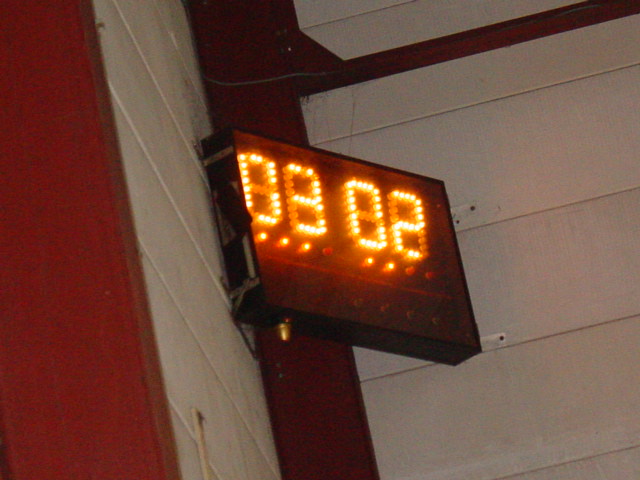This color photograph captures a corner of a space, which could be either an interior room or an exterior alcove. The walls are paneled horizontally and are painted a light dusty pink. Prominently positioned at the corner of the image is a wooden beam, which is stained a deep maroon color. Mounted midway on the wall, there's a digital display with large square dimensions. The display features light yellow numbers against an amber background, reading "8802."